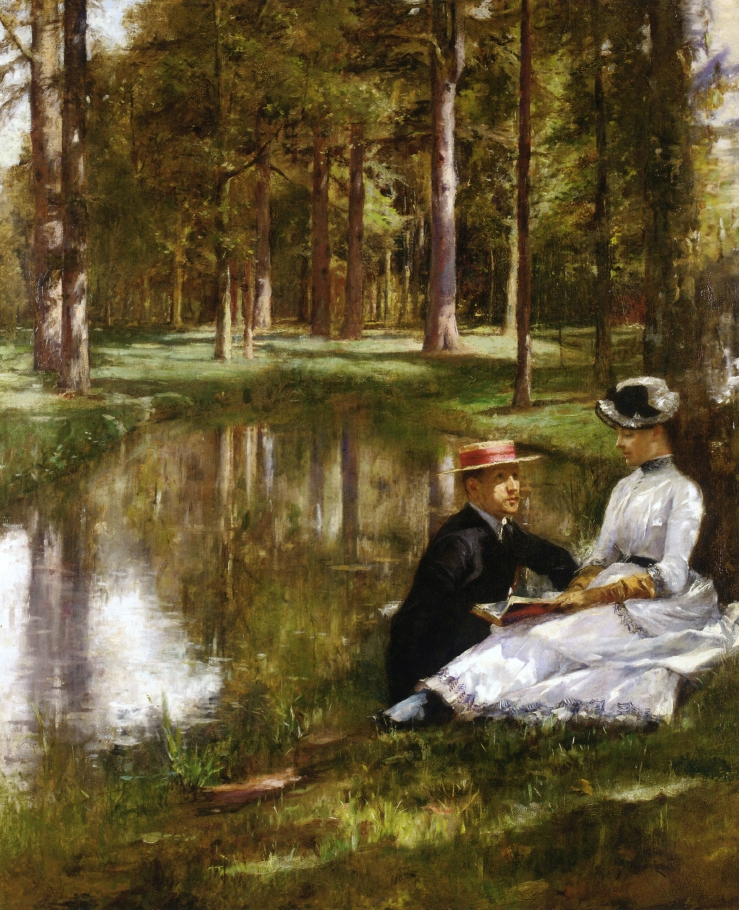In this oil painting set in the style of Monet, titled "Reading Young Romantic Lovers in a Landscape" by Julius L. Stewart, a serene scene unfolds at the edge of a still pond reflecting the dense forest and bathed in daylight. The foreground features a man and a woman situated beneath a large tree. The woman, seated and leaning against the tree in profile on the left side, wears a white dress adorned with long yellow gloves and dark shoes. Her white hat, embellished with a large black bow, contrasts with her silver boots with dark toes and soles. She is engrossed in a book that rests on her lap.

Near her legs, a man dressed in a dark suit with a white shirt and a tie sits, supporting himself with his arms. His straw hat, adorned with a red ribbon, adds a touch of color to his attire. He gazes up at the woman adoringly, seemingly listening as she reads. The daylight casts patterns of light and shadows across the grassy forest floor and the calm water, enhancing the peaceful ambiance of this romantic, woodland setting. The primary colors in the painting are the greens of the trees, as well as the blacks and whites of the couple's attire.